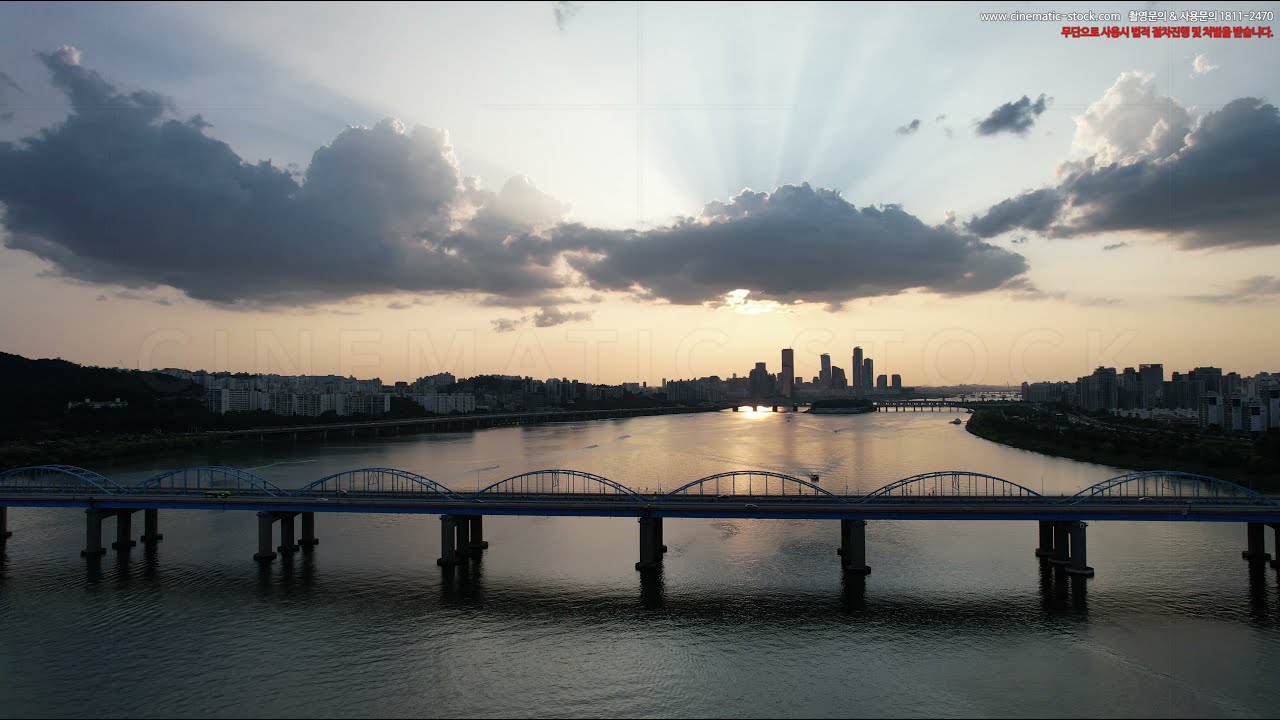This aerial image captures a stunning view of a large river flanked by bridges and a city skyline at sunset. The foreground features a prominent bridge with seven supporting columns rising from the water, connected by elegant curved arches. The bridge is viewed from a low altitude, suggesting the perspective of an aircraft about to land. The scene is enveloped in the warm hues of sunset, with the sky transitioning from pale orange at the horizon to light blue above, punctuated by dark, cumulus clouds. Sun rays pierce through the clouds, casting a golden glow over the cityscape. On the left riverbank, a mix of residential homes and medium-rise buildings dot the landscape, while on the right bank, more medium-rise structures come into view. In the background, another bridge spans the river, adding depth to the composition. The image, marked with a faint watermark reading "Cinemastock" and a URL "www.cinemastock.com" in the top right corner alongside Korean writing, offers a dynamic blend of natural beauty and urban architecture.